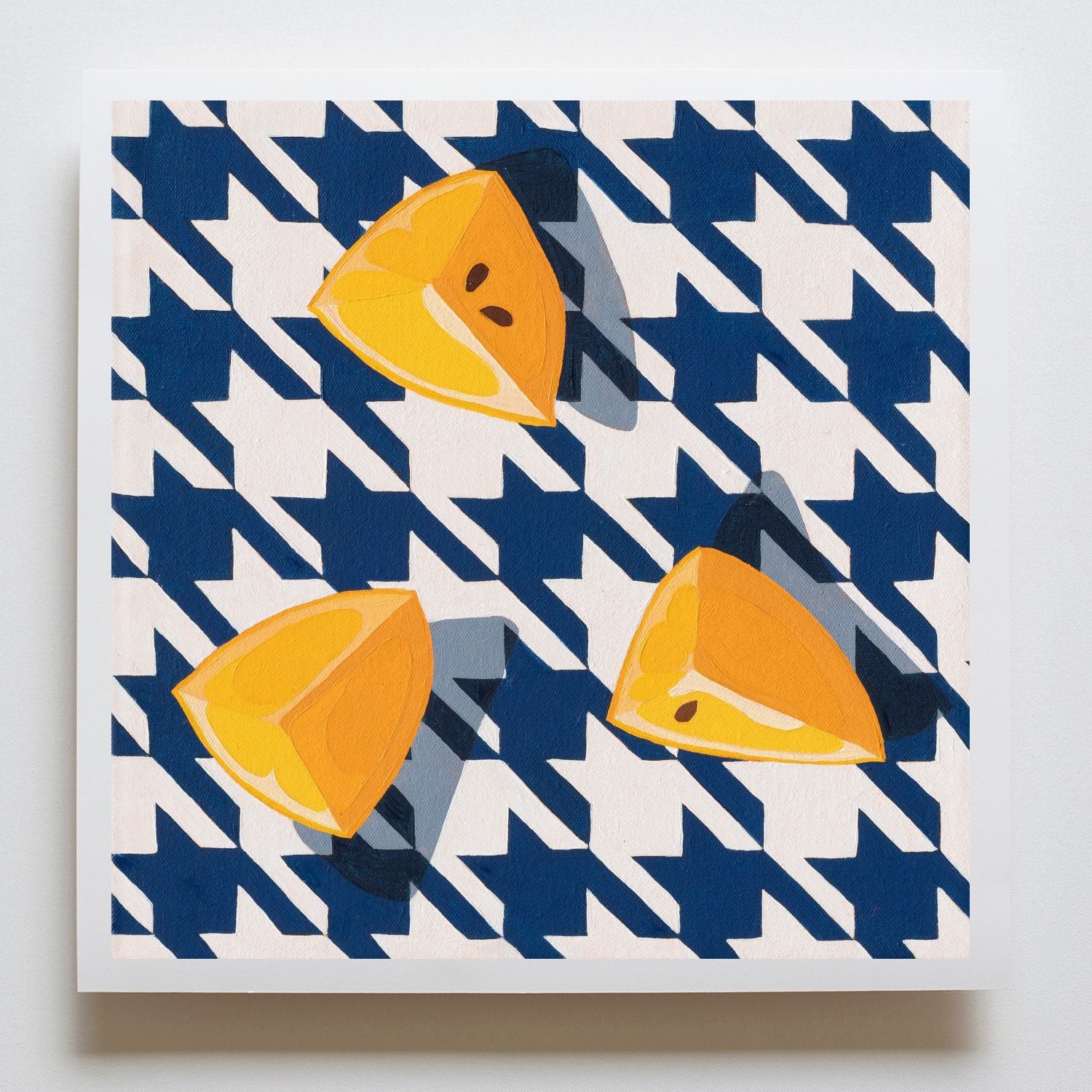This square-shaped image captures a realistic photograph of a wall adorned with a captivating piece of artwork. The piece displayed on the wall features a boldly defined white frame. Inside the frame, a meticulous houndstooth pattern in alternating white and blue sets the backdrop, forming distinctive squarish star shapes. 

Foregrounded against this geometric pattern are three quarter-slices of an orange fruit, painted with a palette of orange and yellow hues. The slices are arranged in a triangular formation, each slice presenting a natural variance; one has two brown seeds, another has one. The painting exhibits a hand-drawn or hand-painted style, adding a personal, textured charm to the composition.

Set against a light grayish-white wall, the canvas creates a soft shadow beneath it, enhancing its prominence. The artwork combines vivid colors and intricate patterns, achieving a harmonious balance that draws the viewer's attention effortlessly.